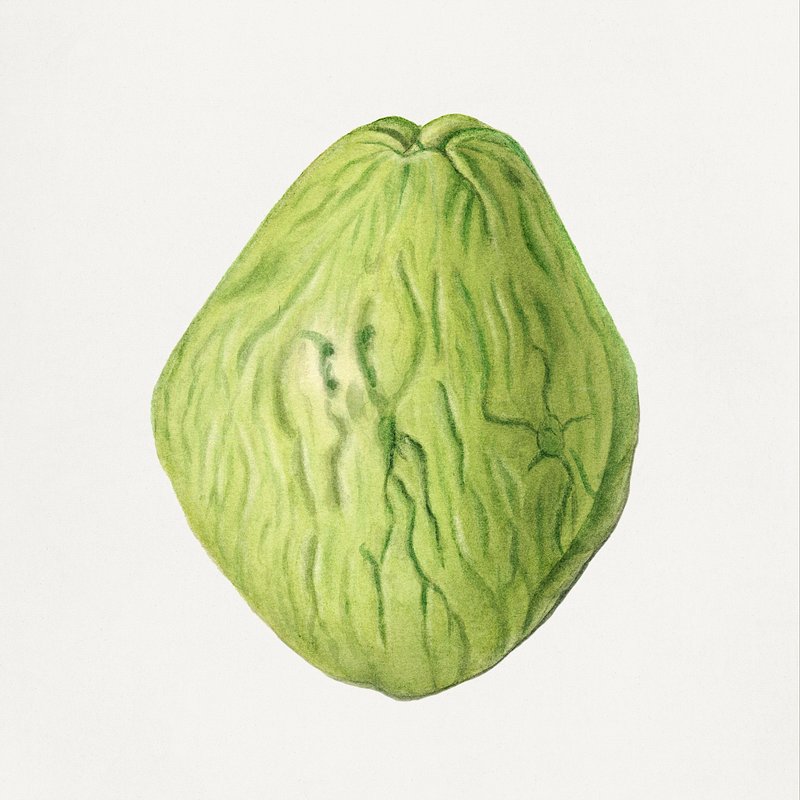The image depicts a unique, green, pear-shaped object that appears somewhat shriveled and is possibly a type of fruit or vegetable. Its light green skin is intricately detailed with veins that stretch out into web-like patterns, and there are numerous non-definitive, vertical, and squiggly lines that add to its texture. Toward the center, there's a patch of white, and at the top, it has small bumps. The object stands vertically on what seems to be a neutral white or light gray background, giving the impression that it’s floating in midair. The image is closely zoomed in, showcasing the distinctive markings and contours of the object, which could be mistaken for a piece of lettuce, cabbage, or a melon.